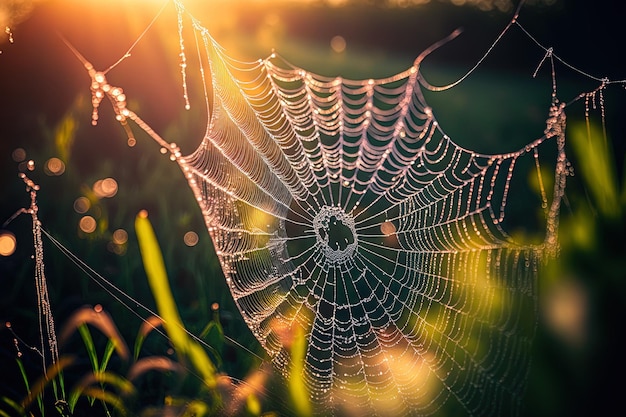This outdoor photograph, taken in the early morning hours, beautifully captures an abandoned and slightly tattered spiderweb adorned with dew droplets. The spiderweb, though partially broken with some large holes, still retains its classic, intricate design with a round center and radiating lines interconnected by circular threads. The sun, shining from the top left, casts a faint glow and sparkle on the dew-laden web, highlighting its delicate beauty. The soft, out-of-focus background features a mix of greenish-yellow and orange hues, with sunlight also illuminating nearby blades of grass and plants. The photo, taken from a low angle within the grass, emphasizes the ethereal and intricate nature of this natural wonder, showcasing Mother Nature's simple yet breathtaking craftsmanship.